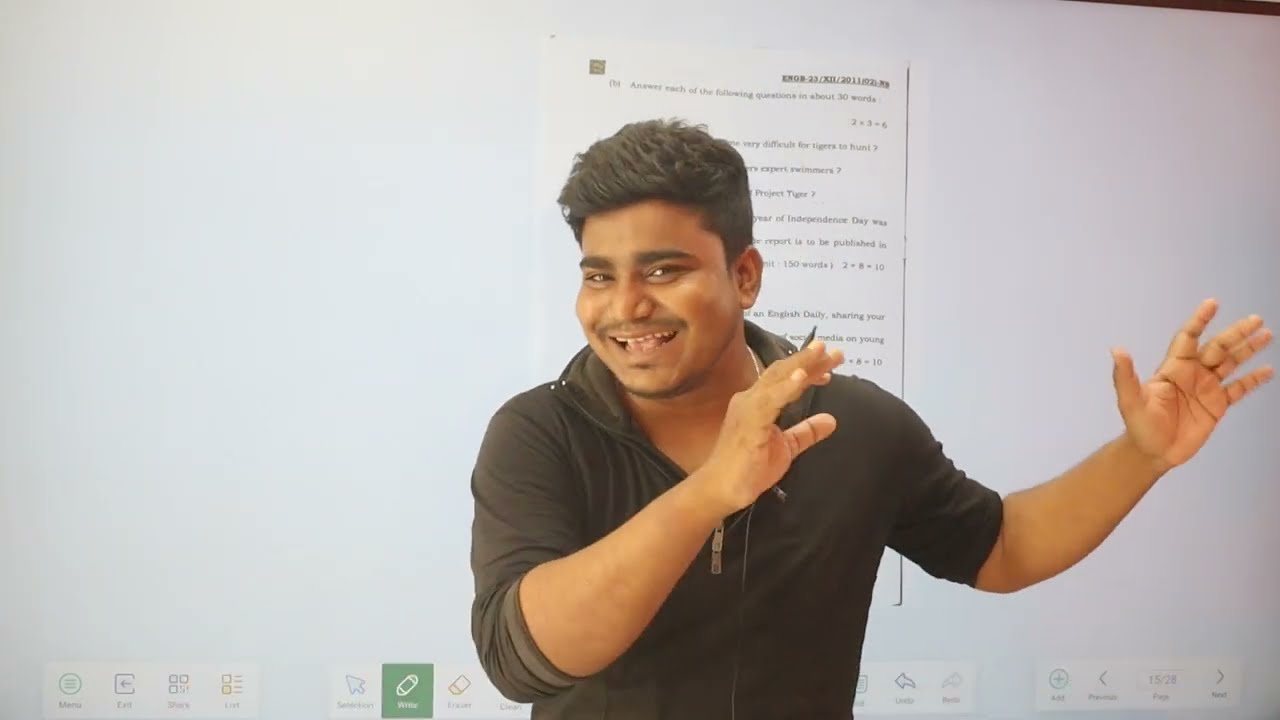In the image, a young Indian man in his 20s stands indoors, appearing to be mid-presentation or perhaps dancing playfully. He has poofy short hair and thin mustache stubble. Wearing a black zip-up sweatshirt with the sleeves rolled up to his elbows, he stands with his hands raised and extended to the right, possibly holding a drawstring from his sweatshirt. He is smiling confidently, suggesting he is either enjoying himself or engaging enthusiastically with his audience. Behind him is a white projection screen displaying black typed text, which may include mathematical equations. Along the bottom of the image are various photo editing tools and computer interface buttons like menu and exit, indicating the scene might be from a video frame or presentation setup.